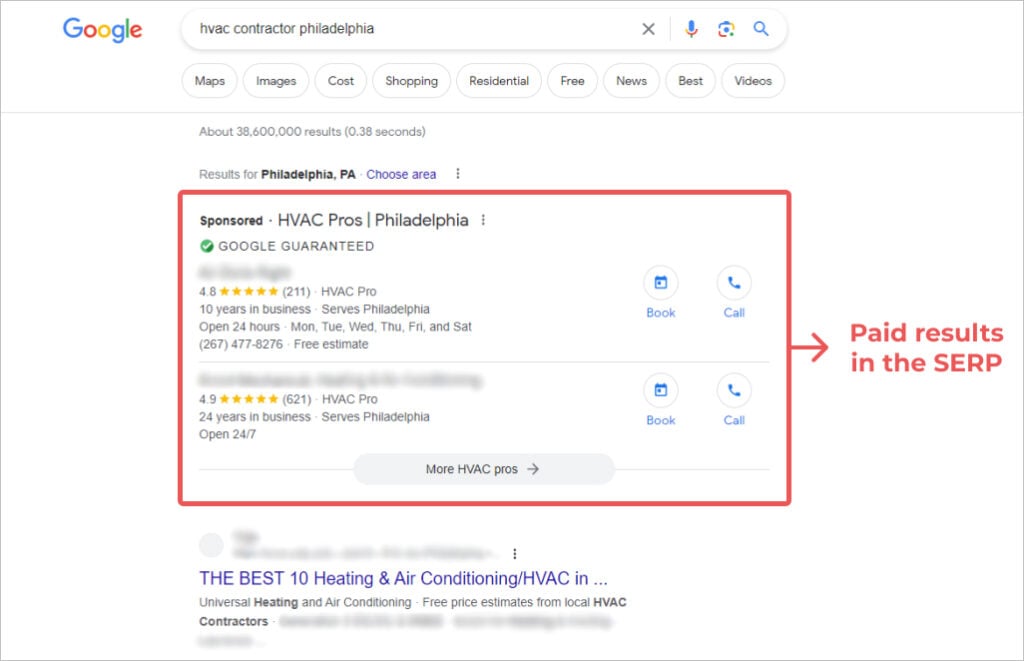Under the category "Websites," the image displays a Google search results page. The Google logo is prominently featured at the top, with its distinctive color scheme: a blue "G," a red "O," a yellow "O," a blue "G," a green "L," and a red "E." Below the logo, the search bar contains the query "HVAC contractor Philadelphia," with an "X" button to clear the search, a microphone icon for voice input, and a magnifying glass icon to initiate the search. Below the search bar, there are several clickable category options including "Maps," "Images," "Cost," "Shopping," "Residential," "Free," "News," "Best," and "Videos." 

Directly beneath these categories, the screen displays the search results summary: "About 38,600,000 results," which seems implausibly high for a local search limited to Philadelphia. It further mentions "Results Philadelphia PA" with an option to "choose area." Next to this, there are three vertical dots indicating additional options. Below these, a "Sponsored" section appears, listing Google-guaranteed HVAC professionals in Philadelphia. The first result shows a 4.8-star rating, and the second result has its name redacted. A red box surrounds these two listings, with a label indicating they are "Paid results in SERP."

Further down, organic search results begin with the heading "The Best 10 Heating & Air Conditioning HVAC."